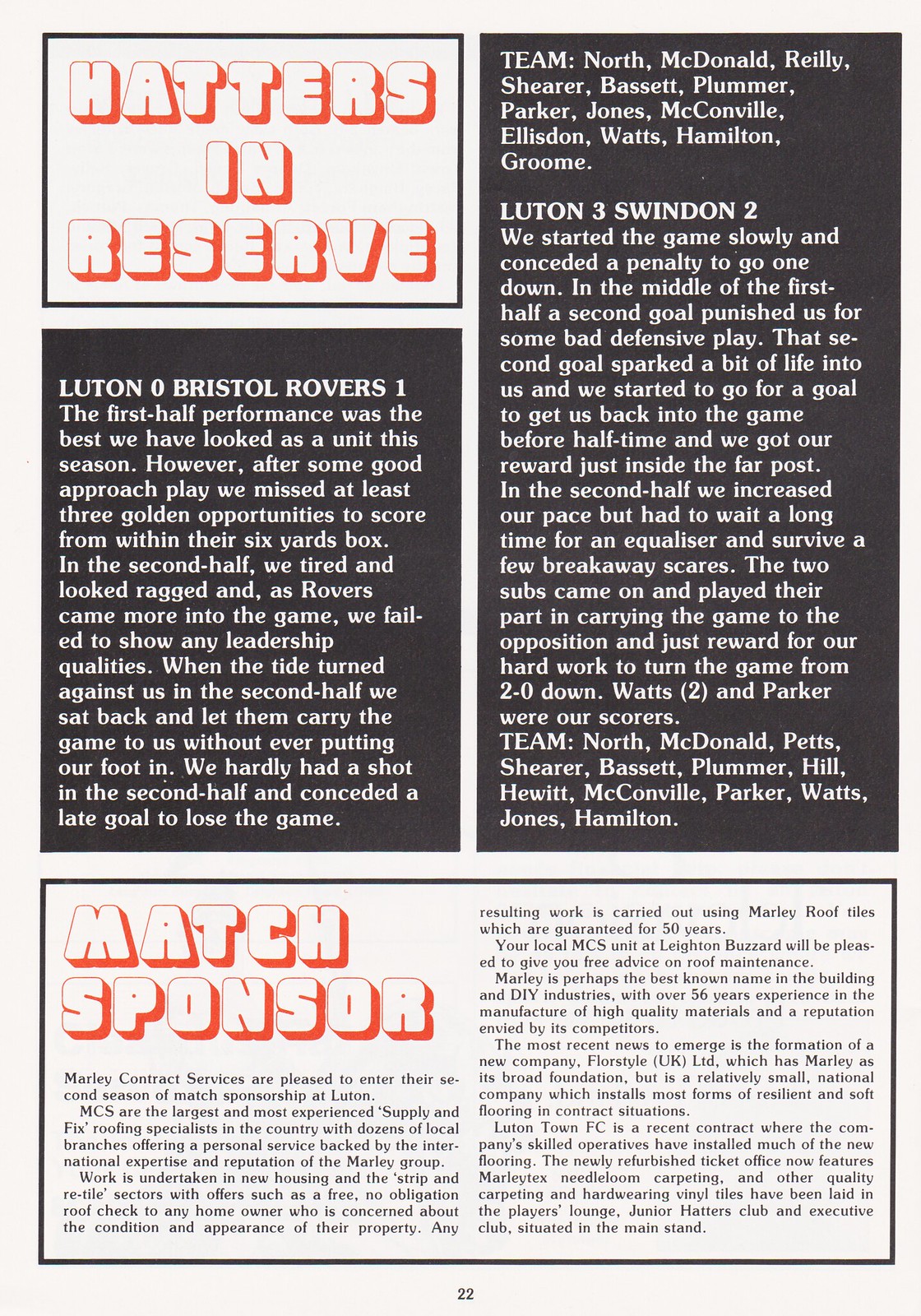The image appears to be a page from an old British football magazine, specifically page 22, featuring extensive match reports and team details. At the top left, there's a white square with white text outlined in red that reads "Hatters in Reserve." Below this, a black text box with white lettering states, "Luton 0, Bristol Rovers 1," followed by a detailed match analysis describing the strong first-half performance and missed opportunities within the six-yard box, leading to a tired and ragged second half without leadership qualities. To the right, another black text box lists team players' names, including North, McDonald, Riley, Shearer, Bassett, Plummer, Parker, Jones, McConville, Elliston, Watts, Hamilton, and Groom. Beneath this, it reads, "Luton 3, Swindon 2," with another detailed game description. At the bottom center, it says "22" indicating the page number. Additionally, at the bottom of the page, there's a white text box bordered in orange that says "Match Sponsor," featuring information about Marley Contract Services.